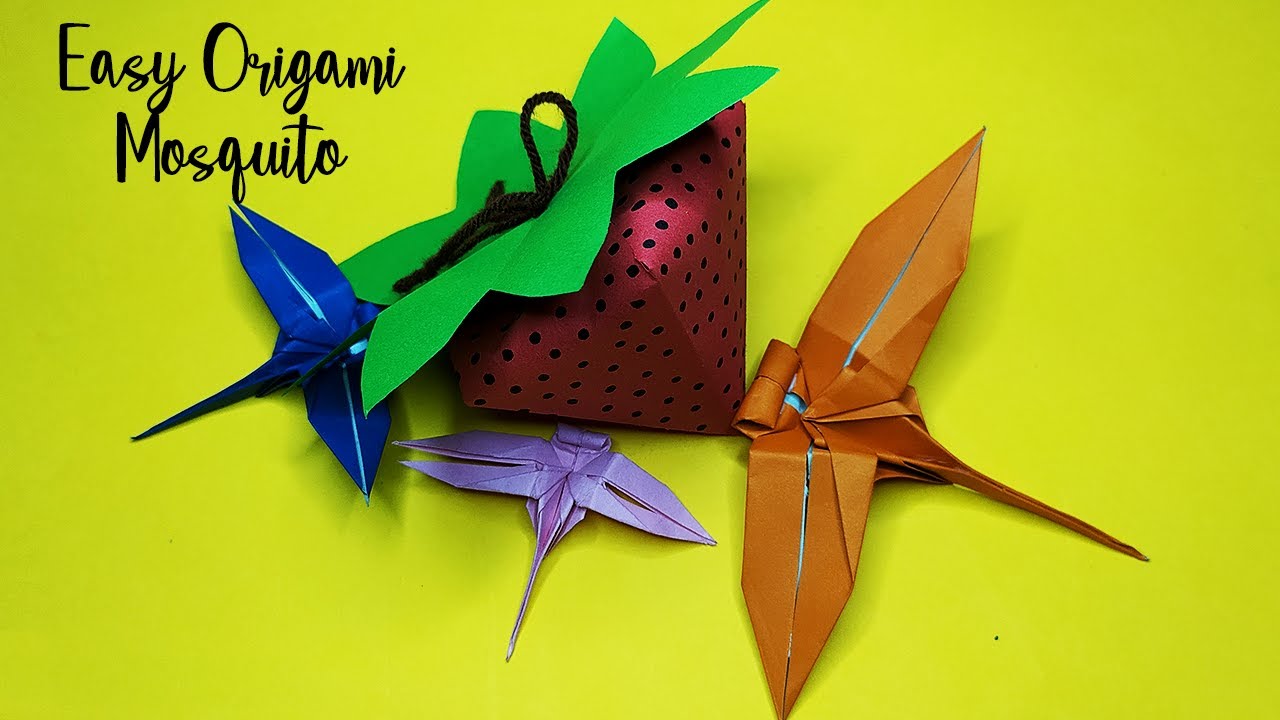The image is a vibrant, horizontally rectangular photograph with enhanced visual effects and a yellowish-green background. The upper left corner features black cursive text reading "Easy Origami Mosquito." Central to the image is a red origami strawberry adorned with black dots and topped with green leaves. Surrounding the strawberry are three origami mosquitoes: on the left is a dark blue, medium-sized mosquito; below and slightly to the right is the smallest mosquito in purple; and on the far right is the largest mosquito, which is orange.